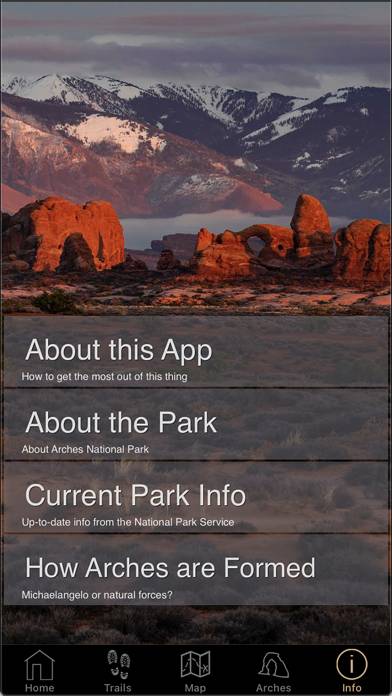This image is a screenshot from an app for Arches National Park, depicting a stunning view of the park during sunset. The arches stand majestically lined up next to each other, bathed in a golden hue from the setting sun. Snow gently dusts the ground, while towering, snow-capped mountains dominate the background. In the foreground, blades of grass are visible, indicating the photographer's proximity to the scene.

Overlaying the image are four translucent white panels with large white text headers and smaller explanatory text beneath each option. The top panel reads "About This App," which likely offers information on how to maximize the app's features. The second panel, labeled "About the Park," provides insights about Arches National Park. The third panel, "Current Park Info," presumably contains up-to-date information from the National Park Service. The fourth panel, "How Arches Are Formed?" explores the geological processes behind the formations.

At the bottom of the screen, five navigation icons are visible: a house icon labeled "Home," two shoe prints labeled "Trails," a folded map with a dashed line and an X labeled "Map," an arch icon labeled "Arches," and a small letter 'i' inside a white circle labeled "Info." The entire image appears to be bordered by a thin, one-pixel black line, which could be part of the screenshot itself.